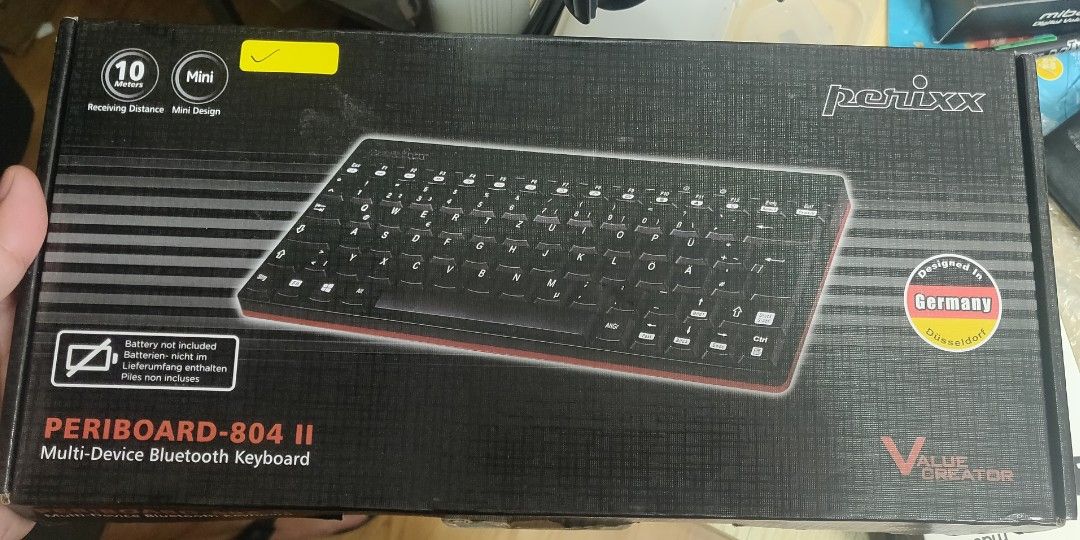The image is a screenshot of packaging for a Peribord 8042 Multi-Device Bluetooth Keyboard. The focal point of the image is a black keyboard prominently displayed in the center of the box. In the bottom left corner, the product name is clearly stated as "Peribord 8042 Multi-Device Bluetooth Keyboard." To the right of the keyboard, a small circle features the German flag, with the word "Germany" written within the circle, indicating the country of manufacture. The top right corner displays the brand name "Perixx," while the bottom right corner bears the phrase "Value Creator." Additionally, the top left corner of the box mentions "Mini," followed by the number "10," although the text beneath "10" is too small to read.